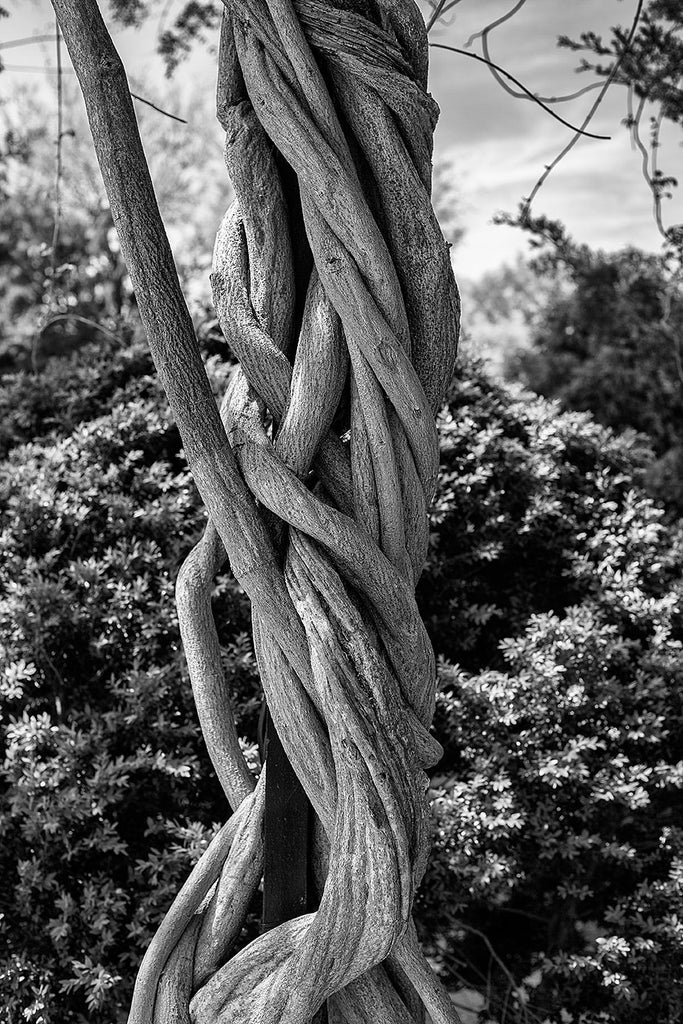A striking black and white photograph captures the intricate beauty of nature with vivid detail. Dominating the center are vertical vines, their complex intertwining reminiscent of braided tree branches, extending from the top to the bottom of the frame. Each vine twists around and beneath the others, creating an elaborate and captivating pattern. On the bottom left, a small section of a black square pole is just visible, offering a stark contrast to the natural forms surrounding it. Behind the twisted vines, lush, leaf-filled bushes create a dense backdrop. Among the vines, a singular branch distinctively extends outward from the center, rising at an angle towards the top left corner of the image. The background is softly framed by a cloudy sky, adding a moody and contemplative atmosphere to the photograph.